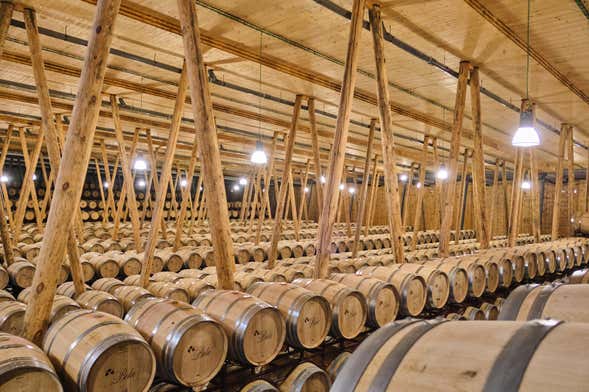The image captures an expansive, cavernous distillery warehouse, showcasing an impressive and seemingly endless array of wooden barrels neatly arranged on their sides. These barrels are meticulously stacked in multiple rows and columns, creating towering horizontal layers that stretch as far as the eye can see, estimated at around 200,000 barrels. The warehouse is constructed entirely of the same color wood as the barrels, giving a warm and cohesive aesthetic to the entire scene. 

From an elevated vantage point, the shot reveals the detailed architecture featuring long rows of A-frame wooden pillars that separate the aisles of barrels, extending from the roof down to the floor or to the shelves where the barrels are placed. Simple lights hang down from the wooden ceiling, illuminating the rustic, orderly space with one light positioned in each aisle. 

The barrels are uniform in appearance, each adorned with a logo in elegant script at the bottom. The warehouse embodies a traditional, artisanal feel, accentuated by the pervasive use of wood in every element, from the walls to the roof, creating a grand and orderly sanctuary for the aging of alcohol.